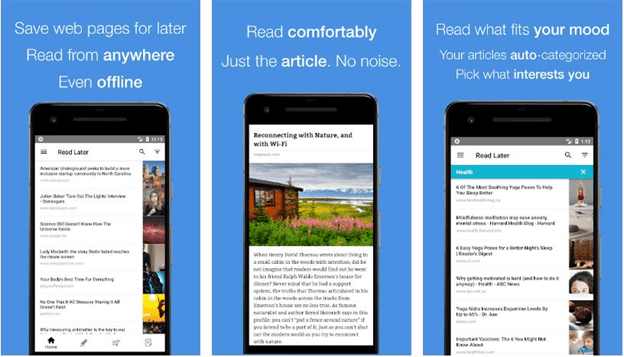This image features a layout with text and three pictures of mobile devices, each highlighting a unique functionality related to reading and saving articles. The first picture emphasizes the ability to "Save webpages for later," allowing users to read from anywhere, even when offline. The second picture showcases how users can "Read comfortably," presenting just the article without any distractions. The third picture highlights a feature where users can "Read what fits your mood," with articles automatically categorized to help users pick content that interests them, whether it's reconnecting with nature or browsing with Wi-Fi for later perusal. The visual elements use a color palette predominantly featuring shades of blue, white, red, green, and brown, contributing to a cohesive and visually appealing design.